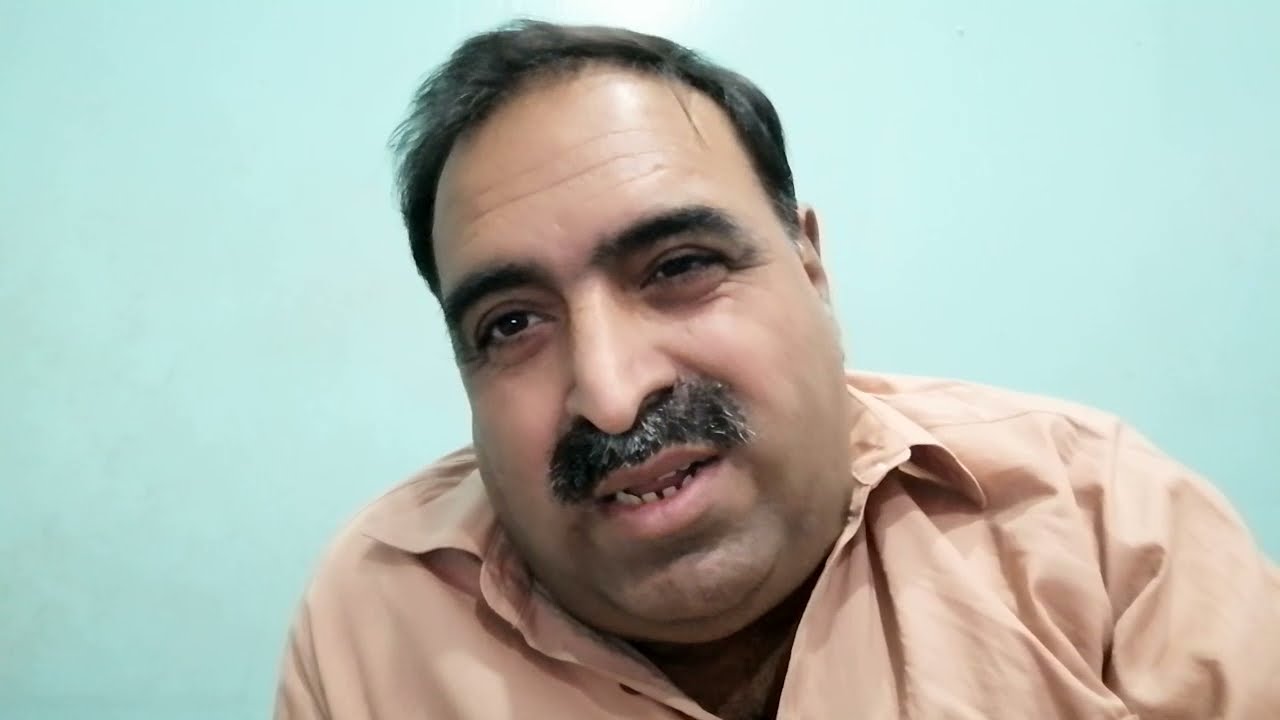The image depicts a man of Indian descent seated against a light teal, almost sky blue, background. The photo, which has a wide rectangular format, captures him from the shoulders up, and he appears slightly offset to the right of the frame. His grimace reveals teeth that are somewhat spaced apart, and his right eye squints more than the left, giving his face an asymmetrical look. Thick eyebrows frame his expressive eyes. He has light brown skin, a thick dark brown mustache speckled with gray, and short, somewhat balding dark brown hair. His light salmon or pink collared shirt, which is slightly wrinkled and unbuttoned at the top, reveals a possible undershirt beneath. The shirt fits loosely around his neck and shoulders, adding to the casual, unposed nature of the image. Judging from the jowls and roundness of his face, he is somewhat overweight. A subtle white light source is visible at the top center of the frame, adding to the ambiance of the room.